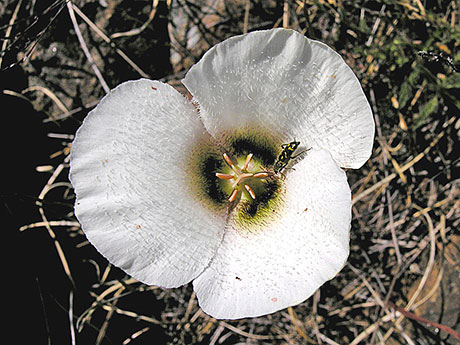The image is a close-up of a white flower with three circular-looking petals, fully opened to showcase its intricate textures and slight wrinkles. The petals are accented with specks of gray and are curved in shape. At the center of the flower, six white spikes, or stigmas, are visible, though there are hues of pale pink, black, green, and orange intermingled. Cast by the Sun, shadows play upon the petals, enhancing their details. Perched close to the pollen-rich center is a long black and yellow insect, possibly a fly. The flower stands out against a backdrop of green leaves, brown twigs, and dead grass, painting a detailed and vibrant scene.